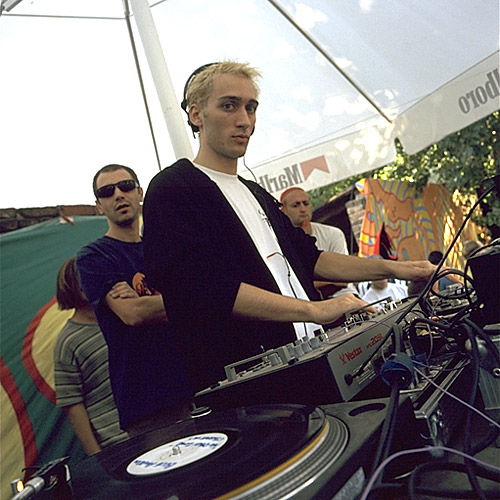The image features a DJ with short, spiky blonde hair and bluish-brown eyes, dressed in a white t-shirt with a black sweater layered over it, the sleeves of which are rolled up to his elbows. He is intently working at a turntable machine, adjusting his equipment while wearing a headset. The DJ is outside under a canopy with a visible Marlboro logo and a yellow flag draped between the sections of the logo. The scene includes a clear blue sky with scattered clouds in the background. Surrounding the DJ are several men, including one in a blue shirt with sunglasses, another in a gray and white striped shirt, and others in white shirts. The photo, with its square format, captures the lively outdoor atmosphere with the DJ looking directly at the camera.